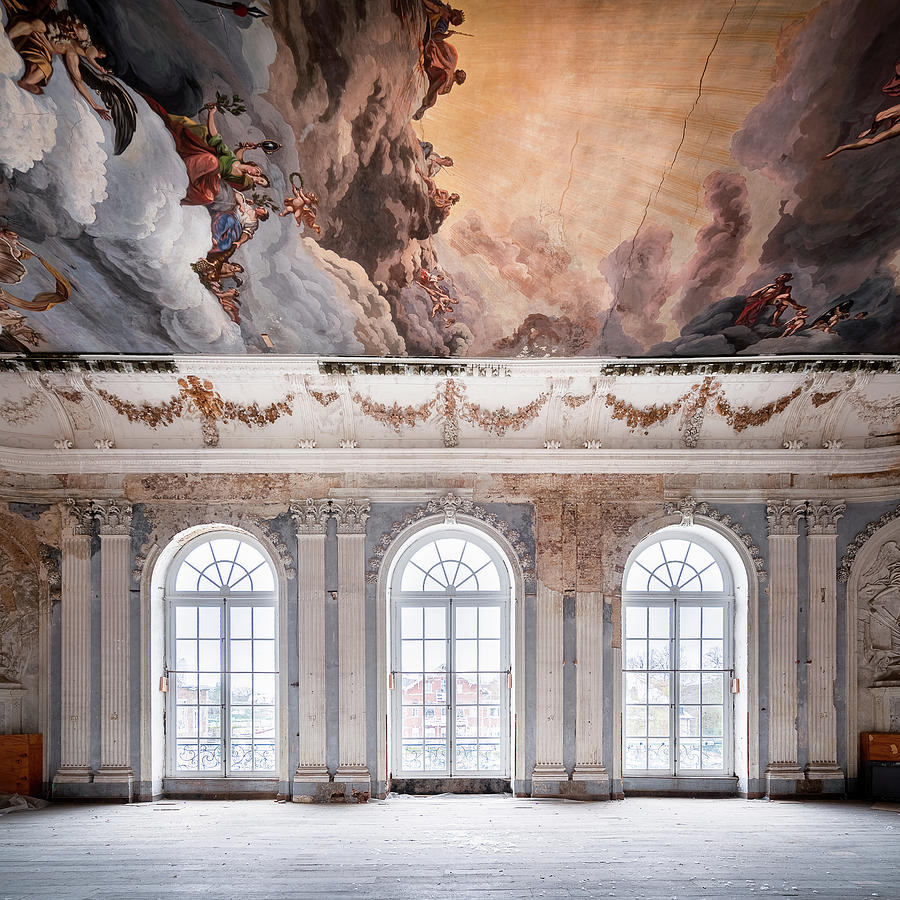The interior of the large building features three prominent, arched, multi-paned windows positioned centrally at the bottom of the image. The upper portion of the windows is adorned with intricate plaster work and painted areas, while Corinthian-topped columns in relief flank the sides. Dominating the upper section of the image is a vivid mural that seems to depict a heavenly scene with clouds turned on their edge. Within the clouds, numerous figures draped in green and orange populate the left side, seemingly floating among ocean waves or clouds. A radiant orange area suggests the morning sun's rays, illuminating the scene. Some figures, possibly monks, sit bareheaded on rocks, while others against a purple backdrop to the right appear ambiguous and mystical. Angels flying above and figures with cape-like or wing-like extensions add to the ethereal atmosphere. The foreground reveals a deteriorated white building with a decorative trellis and aged, circular windows, suggesting an ancient, almost sacred place. The floor beneath is composed of gray wood, enhancing the historical and weathered ambiance of the scene.